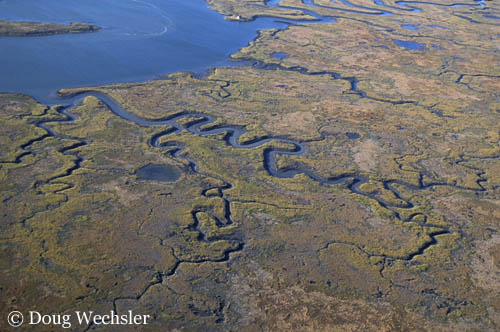This aerial view captures the striking contrast where land meets water, showcasing a detailed marshland with intertwining rivers and streams. The image, a horizontally aligned rectangle, prominently features a large blue body of water in the upper left corner, from which numerous channels and deltas snake through the landscape like winding serpents. The land itself appears as irregularly shaped, puzzle-like pieces, predominantly displaying hues of green and brown. These colors hint at a marshy or swampy terrain, with green grasses or algae interspersed with patches of brown dirt. A notable feature includes a larger water body resembling a pond situated in the central area, while smaller streams crisscross the scene. No human structures are visible, emphasizing the untouched natural setting. The lower left corner of the image bears a white copyright symbol followed by the name "Doug Wechsler."